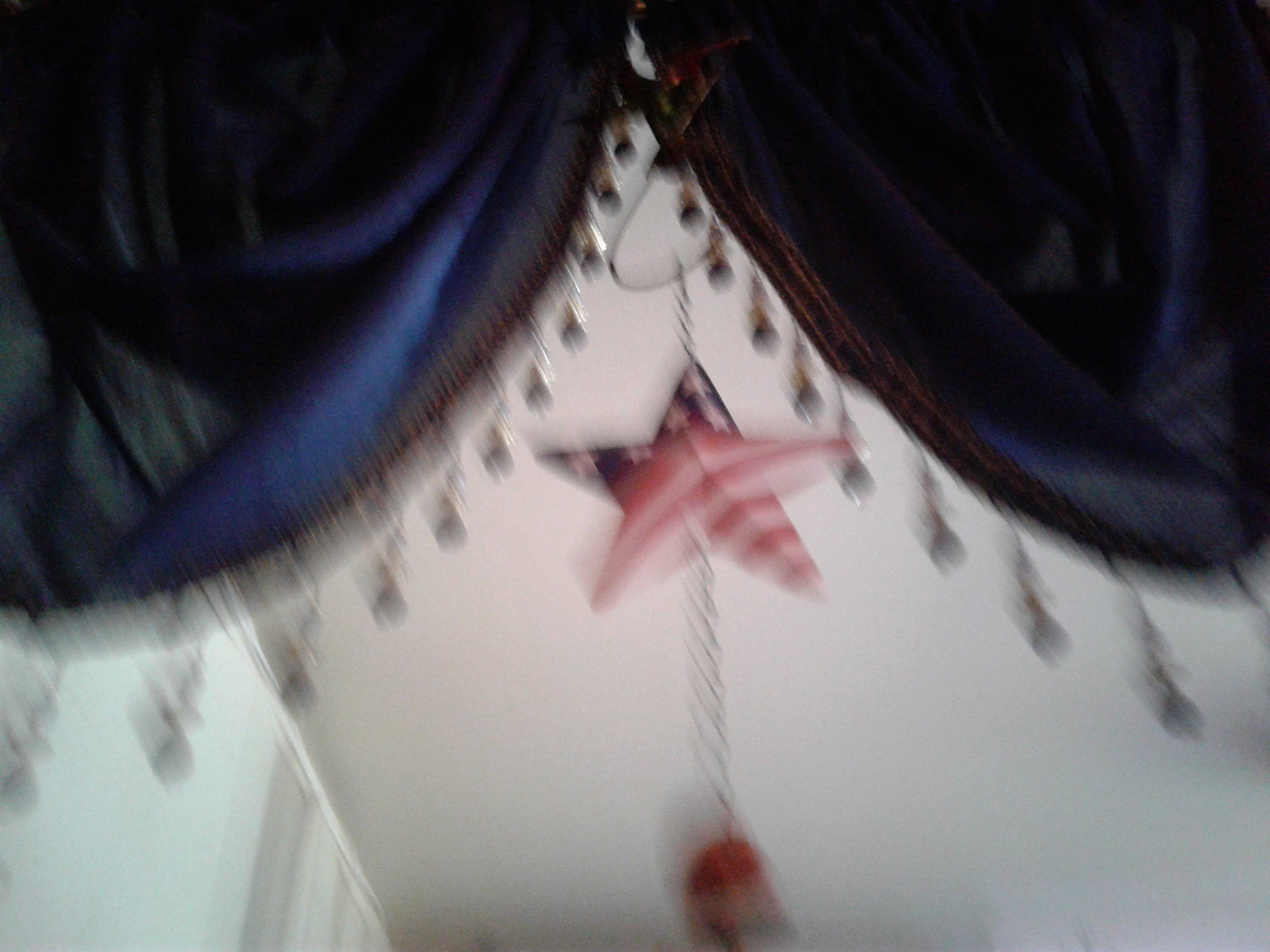The blurry photograph depicts a pair of blue curtains that drape elegantly from the top edge, extending down to form circular patterns at the corners and along the sides. The soft blue fabric is adorned with dangling ornamentation, featuring metallic bristles, beads, and little bells or charms that line the curtains from top to bottom. At the center hangs a prominent metal star, decorated with American flag colors: the top right and left points are dark blue with white stars, while the bottom three points are painted with red and white stripes. From the middle of the star hangs a chain or pull tab, with a reddish hue and possibly yellowish or beige details, though it's indiscernible due to the overall blurriness. Behind the curtains, a slightly tinged light blue wall and a white ceiling are faintly visible. The image’s lack of clarity suggests it was captured with a shaky hand, resulting in a general blur across the entire scene.